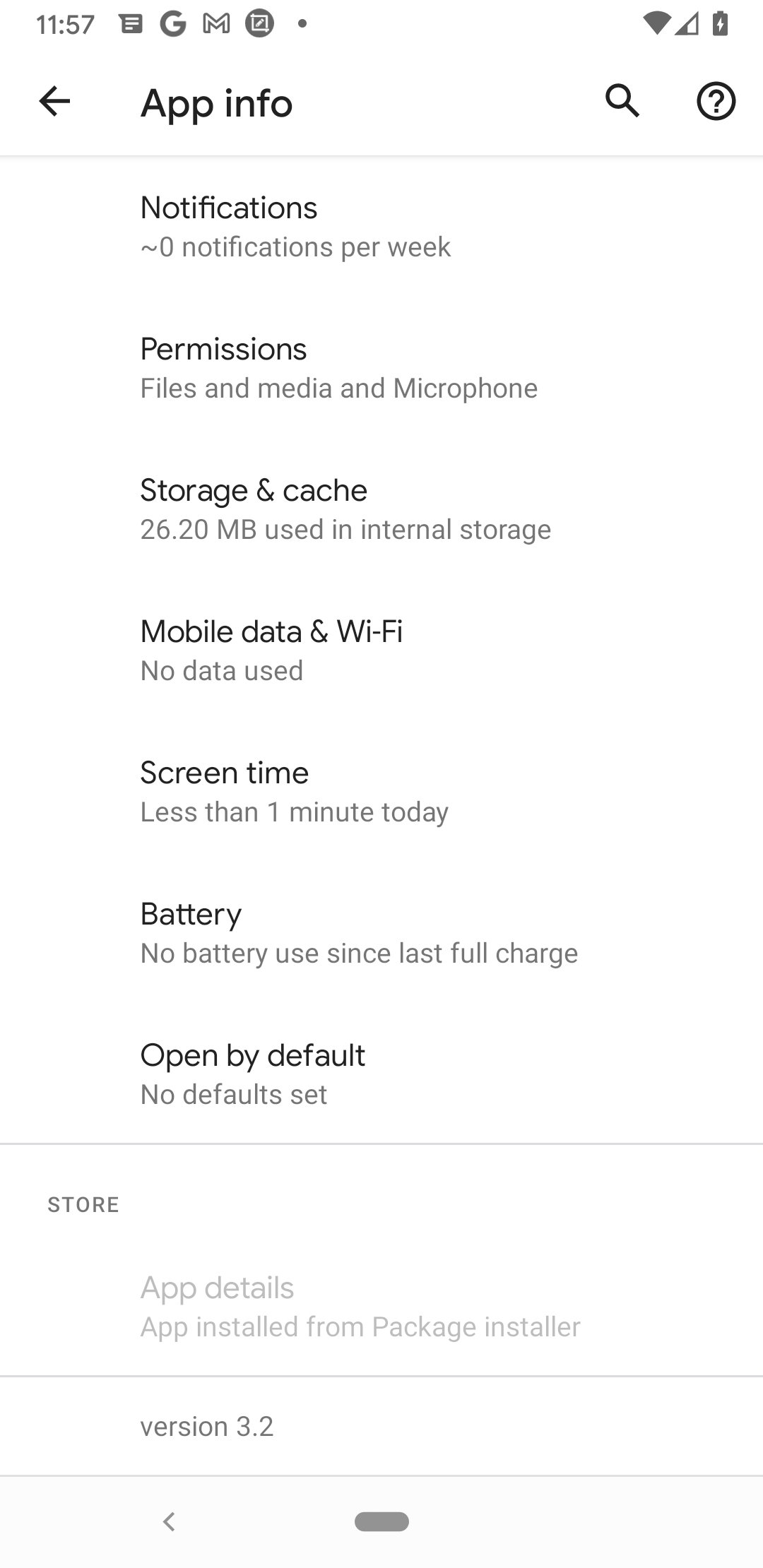The image is a screenshot of a phone displaying app information. 

In the top left corner, the time displayed is 11:57. The status bar shows various icons, including the Gmail app, indicating notifications from Gmail. The phone's reception is weak, although the battery is fully charged. 

Currently, the screen shows the 'App Info' section of a specific application. At the top right, navigation options allow the user to go back, pull up a search bar, or add a question bubble.

The information is listed in a light black, thin font, with subcategories in gray. The details are as follows:

- **Notifications**: Zero notifications per week.
- **Permissions**: Access granted to Files and Media, and Microphone.
- **Storage and Cache**: 26.20 megabytes used in internal storage.
- **Mobile Data and Wi-Fi**: No data used.
- **Screen Time**: Less than one minute today.
- **Battery**: No battery usage since the last full charge.
- **Open by Default**: No default set.

Separated by lines, additional details are listed:

- **Store**: App details indicating the app was installed from the package installer and is currently on version 3.2.

This detailed description suggests that the user is reviewing the information of a recently installed application.